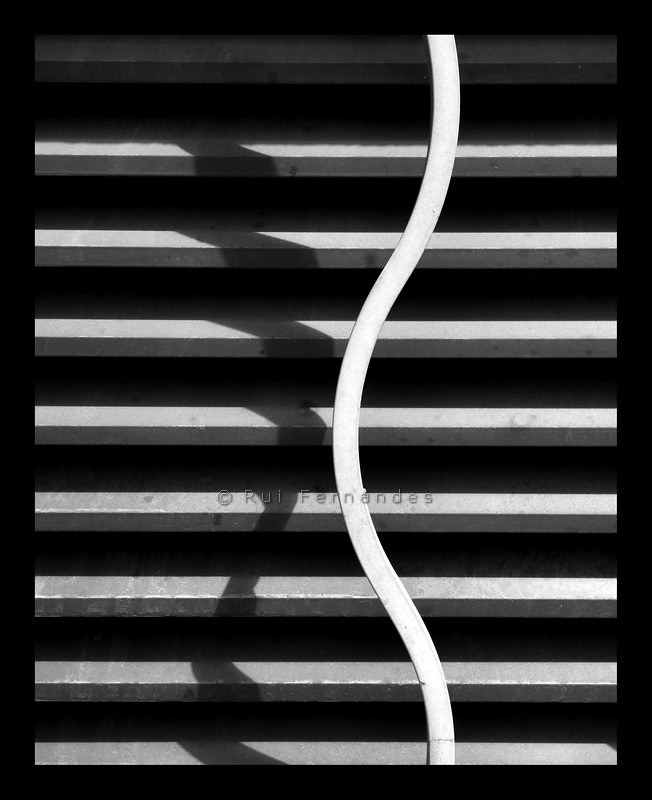In this black and white photograph, horizontal metallic beams or possibly slats, resembling window lines or a vent, form the background. Superimposed over these horizontal bars is an undulating vertical stripe, a white curved bar that runs from top to bottom, casting a distinct shadow onto the bars behind it. The image is bordered by a black frame that marks its boundaries. In the center, there is a faded watermark with copyright text reading "Rui Fernandes," including a circled "C" indicating a copyright symbol. The juxtaposition and shadows in the image create an intriguing and abstract pattern, leaving the precise nature of the objects open to interpretation.